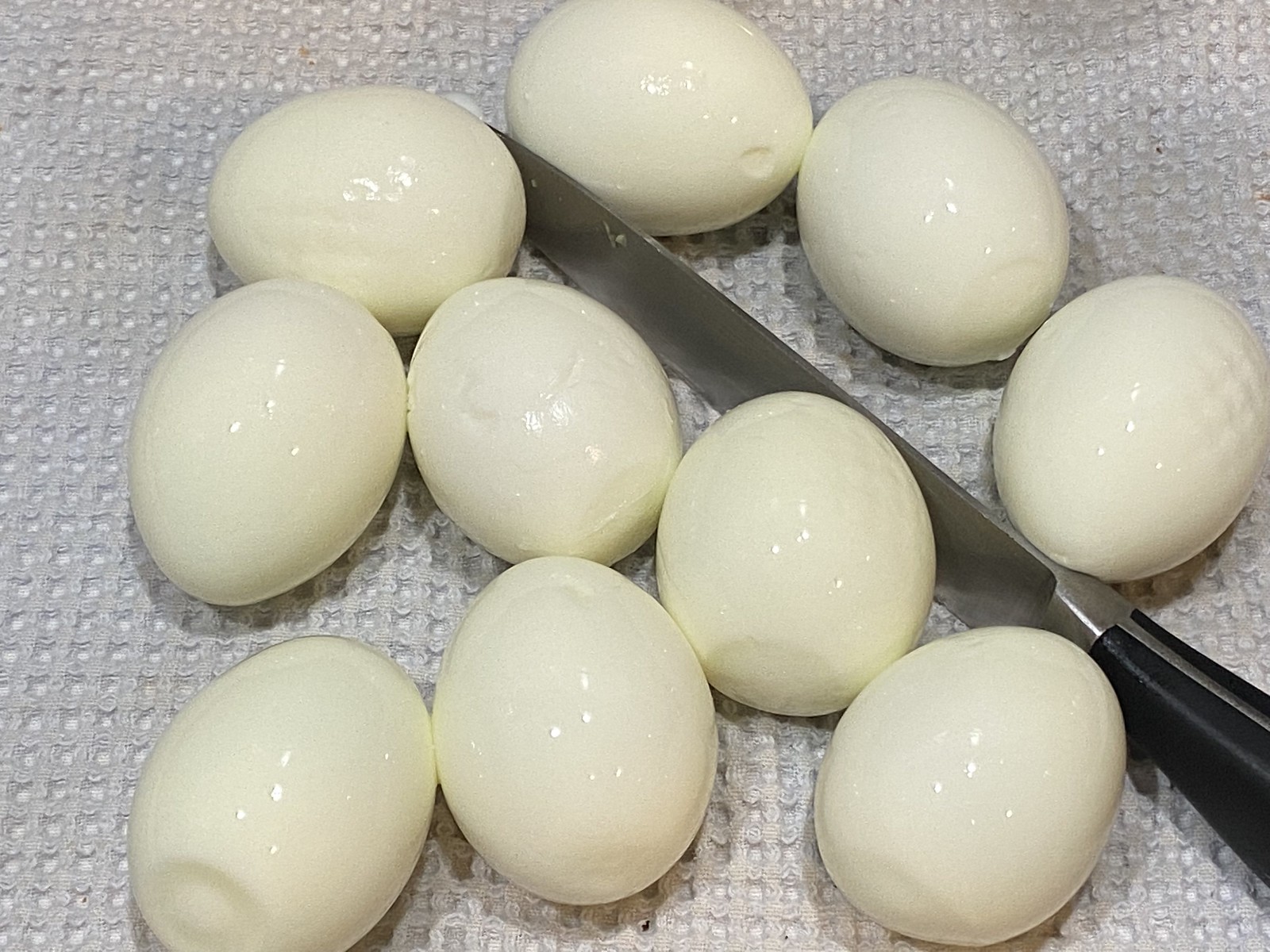In this vivid photograph, ten freshly boiled eggs, with their glistening white surfaces fully de-shelled, are artfully arranged on a waffle-patterned white tea towel, filling the entirety of the background. Three of the eggs occupy the top right corner, while the remaining seven cascade towards the bottom left corner. Dominating the center of this arrangement is a long, sleek stainless steel knife with a black handle. The knife rests on its side, its blade facing downwards, stabilized by the surrounding eggs, a few of which lean against it. The composition highlights the contrast of the smooth eggs against the metallic sheen of the knife and the textured fabric beneath, creating a striking and detailed scene.